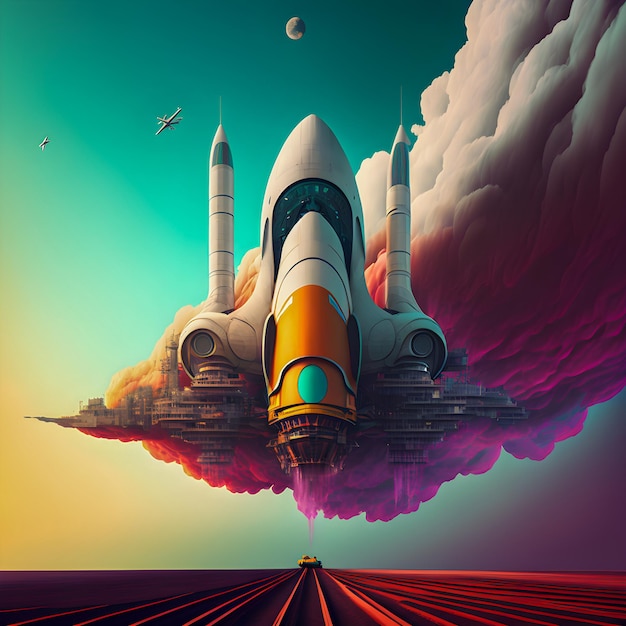The image depicts a highly detailed, futuristic, and somewhat surreal scene featuring a colossal, artificial intelligence-generated spaceship or floating city. This massive structure is propelling itself above a desolate, dirt-filled field, stretching towards a very clear, blue sky. The spaceship appears to be emitting vast amounts of energy, resulting in a gigantic plume of smoke that transitions in color from white to dark purple, blue, pink, and yellow, creating a dramatic visual effect.

The structure has two prominent control centers, resembling silos or landing pads, each topped with rockets bearing large blue windows and needle-like points. The central part of the spaceship has a distinctive large orange nose with a blue dot, transitioning to a whitish gray and ending in a dark bluish-green window. The horizon comprises the bottom eighth of the image, showing reddish-brown furrows that disappear into the distance. At the horizon's center, there is an unclear object.

The surrounding cloud gets denser and darker towards the right and lighter as it ascends. Above, two smaller planes are visible in the sky, one clearly defined and the other more distant. Dominating the center of the sky is a circular moon-like disc, adding to the fantastical ambiance of the scene. The overall depiction is highly imaginative and appears highly unrealistic, reflecting a blend of detailed technological elements and artistic creativity.